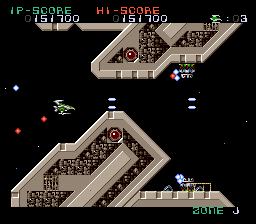The image appears to be a snapshot from a classic arcade or old Atari-style video game, resembling an 80s or 90s side-scrolling space shooter. The background is entirely black, creating a striking contrast with the vibrant elements of the interface. At the top left, in green text, "1P-SCORE" is displayed, directly followed by a high score of "151,700" in white digits. The same high score is echoed in the center-top with the label "HIGH-SCORE" in red. On the top right, a small green spaceship icon is accompanied by the indicator "03" in white, signifying the remaining lives.

In the central part of the image, there are two large tan-colored geometric shapes that appear to be fragments of a space maze or station, filled with intricate gray and brown stone-like walls. The upper shape contains a red eye-like feature and reveals cybernetic innards through window-like openings. Scattered around the shapes, several green and silver spaceships maneuvering from left to right are visible, with two of them positioned underneath the top tan shape and one on the far right of the bottom tan shape. The spaceship on the left-middle is noticeably firing lasers, highlighted by two protruding red beams, amidst red stars and stray blue-white dots in the background, which could represent stars or projectiles.

In the bottom right corner, against the continuous black backdrop, "ZONE" is displayed in green text followed by the letter "J" in white. Here, additional miniature elements like blue lines and cannon-like structures suggest active combat, reinforcing the image's engaging space battle ambiance.